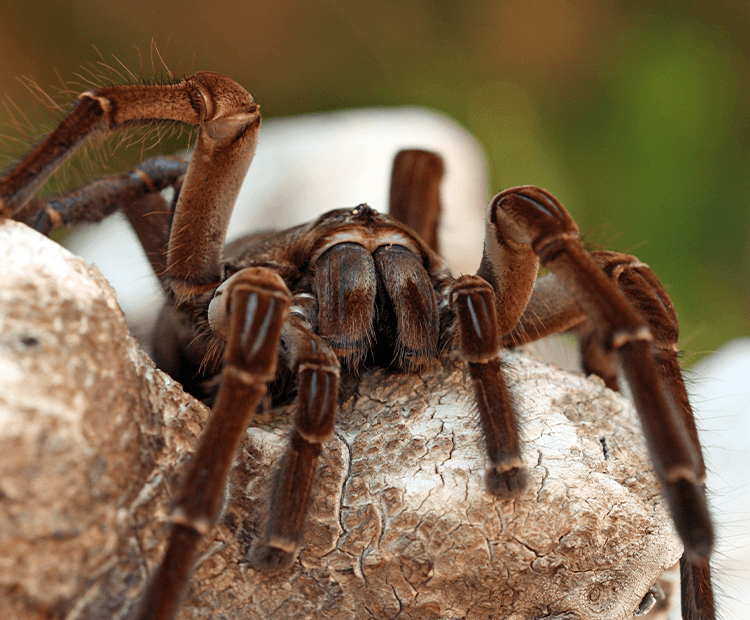This close-up colour photograph captures a large tarantula, exhibiting a dark brown to reddish hue, perched atop a light tan to brown, crackle-textured stone, possibly aquarium or tank decor. The tarantula's large fangs are prominently visible, and the vivid detail of its long, hairy legs and talon-like appendages, which grasp the stone, are in sharp focus. Although only a part of the spider's body is visible, several fine details, including its almost discernible eyes and cute little paws, are noticeable. The blurred background features hues of green, white, and brown, with a distinct roundish white object creating a striking contrast. Hints of additional white and brown objects appear in the right and lower corners, framing the terrifying yet fascinating scene.